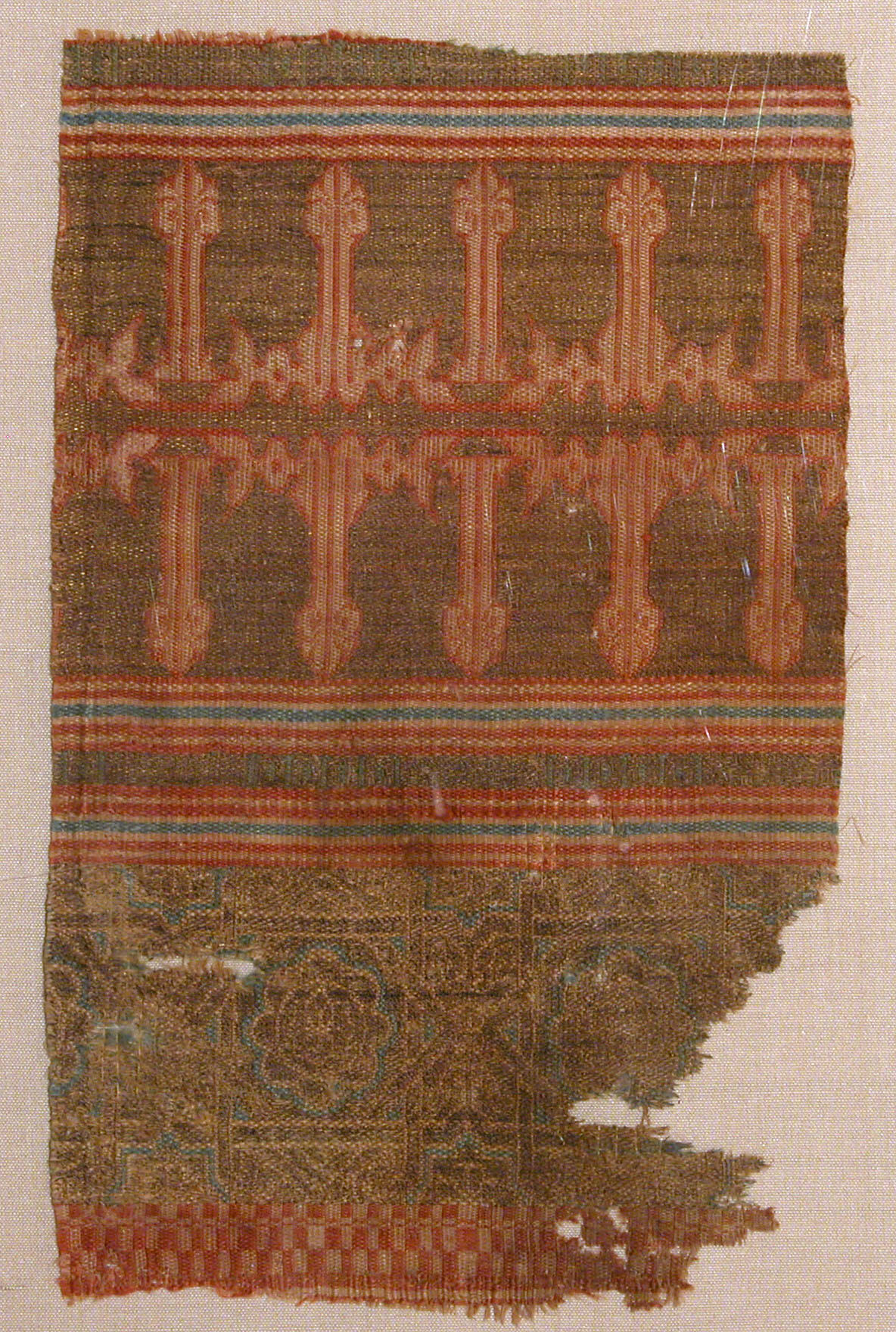The image depicts an ancient, decaying textile piece displayed on a white linen background. The rectangular fabric is primarily burnt orange with various shades of brown interwoven throughout. At the bottom, it features an intricate, albeit deteriorating, ornate design, partially obscure due to its age. A checkerboard pattern interlaced with blue and brown dominates the lower section, enhancing the antique's faded elegance. Above this, a multicolored banner runs horizontally with vibrant reds, blues, whites, and yellows still visible, contributing to the tapestry's ornate designs. This intricate detailing continues upwards, with another multicolored banner leading to more intricate patterns, including stripes and larger, floral motifs in the top half. Notably, the bottom right corner is missing, a testament to the textile's ancient and fragile condition.